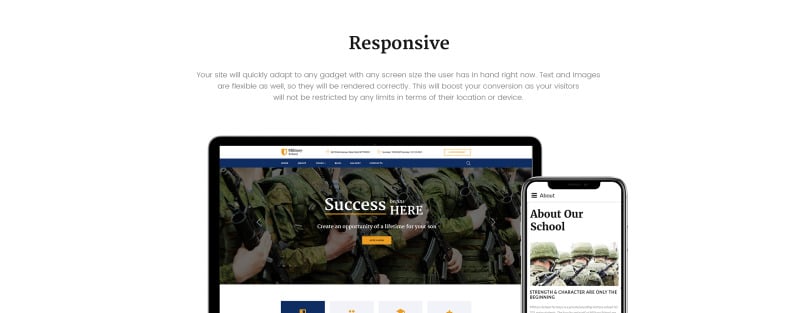The image features a clean, white background with prominent black text centered at the top, which reads "Responsive." Beneath this, in lighter gray text, are the words: "Your site will quickly adapt to any gadget with any screen size the user has in hand right now. Text and images are flexible as well, so they will be rendered correctly. This will boost your conversion as your visitors will not be restricted by any limits in terms of their location or device."

Below the text, there is a generic laptop screenshot with a black bezel. The screen displays a white banner at the top featuring some black text, along with an image of individuals in camouflage uniforms holding black guns, suggesting a military context. Above the image, in white text, the word "Success" is visible, though partially obscured by another word.

To the right of the laptop image is an iPhone displaying a webpage with a white background and black text, which reads "About Our School." This further implies that the website being advertised is likely for a military school. A yellow button is present underneath the text on the laptop screen, drawing attention as a call-to-action.

The overall composition of the image suggests a responsive design that works seamlessly across various devices, emphasizing the adaptability and user-friendliness of the website, which in this case, appears to be a military school.